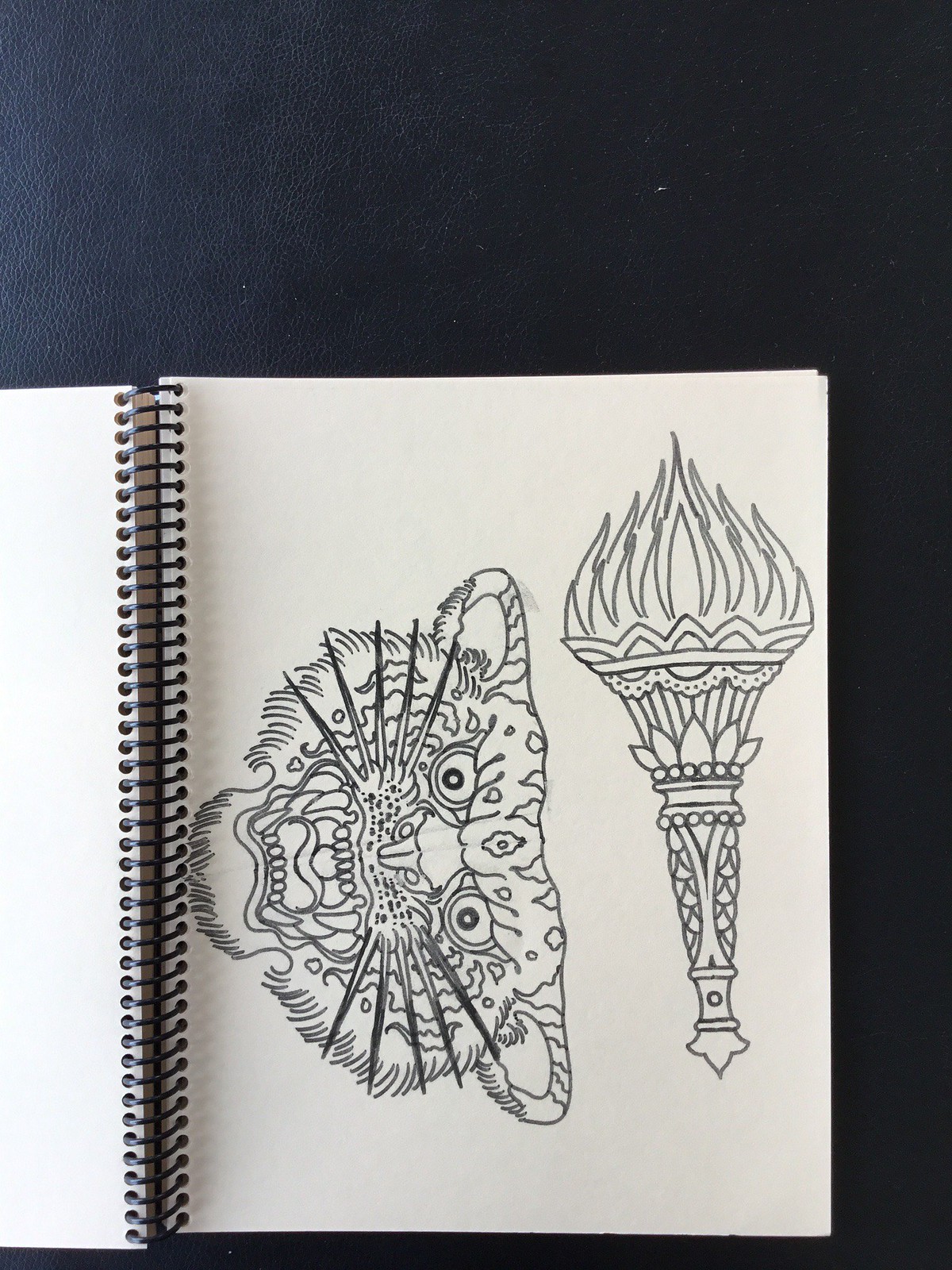In this photograph set against a near-black background, an open spiral-bound notebook takes center stage. On the left page, which is stark white, sits an intricate pencil or marker drawing of a tiger's face. The tiger appears ferocious, its mouth agape, revealing sharp fangs flanked by long whiskers. Its eyes, dark and intense, convey a palpable sense of anger, and speckled patterns mark the top of its ears. Adjacent to this, on the slightly off-white page to the right, is a detailed illustration of a torch. The torch is adorned with elaborate designs consisting of flowers, dots, and lines, and it supports a fierce flame that rises in sharp, vivid peaks. The intricate artistry of both the tiger and the torch captures attention, vividly contrasting against the dark backdrop.